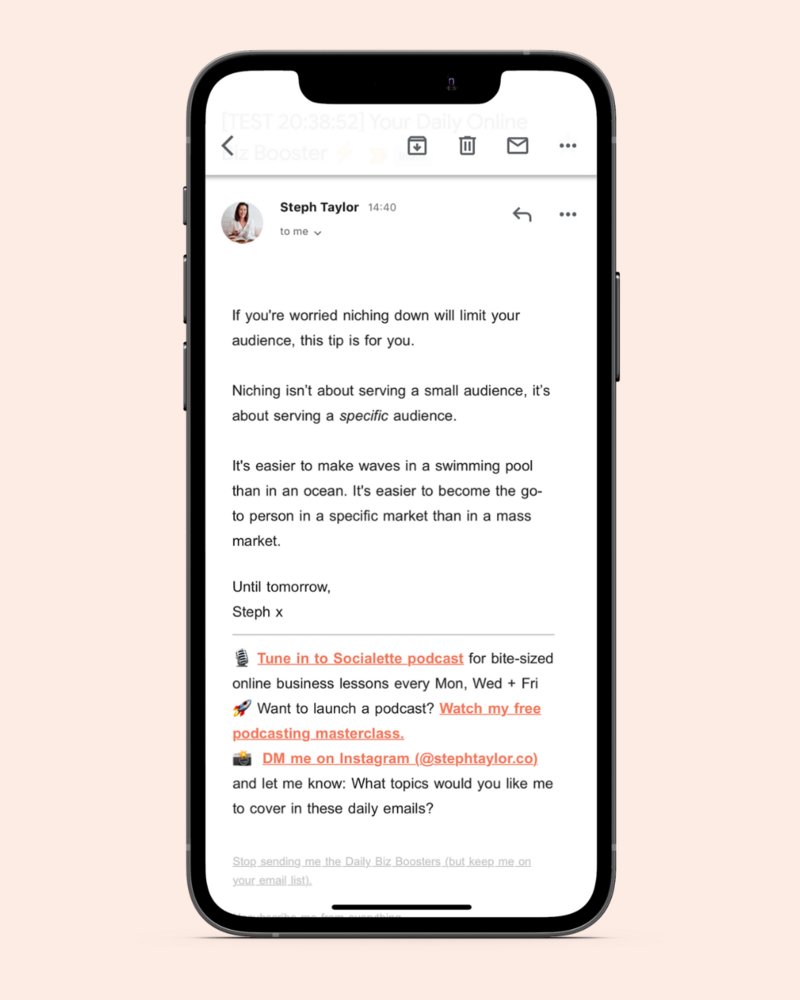The image depicts the entire interface of a cell phone, showcasing both its physical and digital aspects. The phone has a black outline, with three physical buttons on the left side and one on the right side. The digital interface displayed is a fully detailed email screen, not merely a webpage.

At the top of the screen, there are several functional icons, including a back button, a download button, a trash button, a mail button, and a menu represented by three vertical dots. These icons are separated from the email's content by a horizontal bar.

The email itself is from Steph Taylor, received at 14:40. Steph Taylor's profile picture is visible, and the email is addressed to the viewer. There is a dropdown menu to view recipient details and a reply button represented by a curvy left arrow. Clicking on the three vertical dots provides additional options such as "Forward," "Reply All," and more.

The email message reads as follows:

"If you’re worried niching down will limit your audience, this tip is for you. Niching isn’t about serving a small audience. It’s about serving a *specific* audience. It’s easier to make waves in a swimming pool than in an ocean. It’s easier to become the go-to person in a specific market than in a mass market. Until tomorrow, Steph x."

Following the email text, there are various clickable links and advertisements to connect with Steph Taylor's content and social media. These include:

- A link to the Socialette podcast for bite-sized online business lessons every Monday, Wednesday, and Friday.
- A link to watch her free podcasting masterclass.
- An invitation to DM Steph on Instagram at stephtaylor.co with topic suggestions for the daily emails.

At the bottom, there is an unsubscribe option in very light print that reads, "Stop sending me the daily biz boosters but keep me on your email list." This allows users to manage their email preferences without fully unsubscribing.